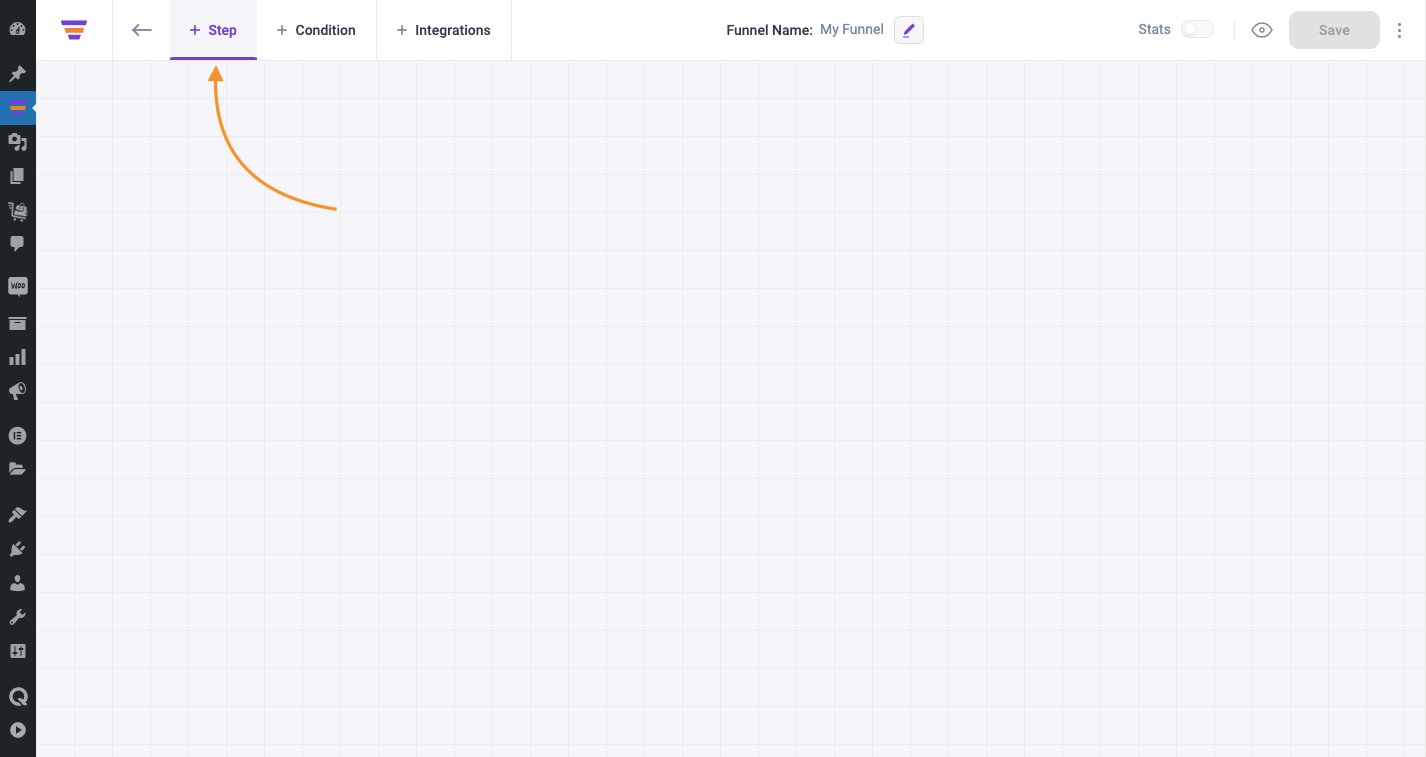On the left side of the image, there is a long black vertical bar featuring various symbols arranged vertically. The symbols include a push pin at the top, followed by a blue square with a pink center, a white square that resembles a book, more white squares further down, and three vertical lines placed beside each other. Continuing downward, there is a paintbrush, a wrench, and at the very bottom, a search icon depicted as a magnifying glass.

At the top of the bar, the word "Step" appears, underlined in purple with a purple plus sign to its left. An orange arrow points upward toward this underlined word. To the right of "Step," the words "Condition" and "Integrations" are displayed sequentially. Approximately three inches to the right of these words, the phrase "Funnel Name" appears, followed by lighter text that reads "My Funnel."

Adjacent to this, there is an image of a purple writing utensil, which could be a pen or pencil. A couple of inches further to the right, the word "Stats" is visible. Finally, at the far right, there is a horizontal box containing the word "Save."